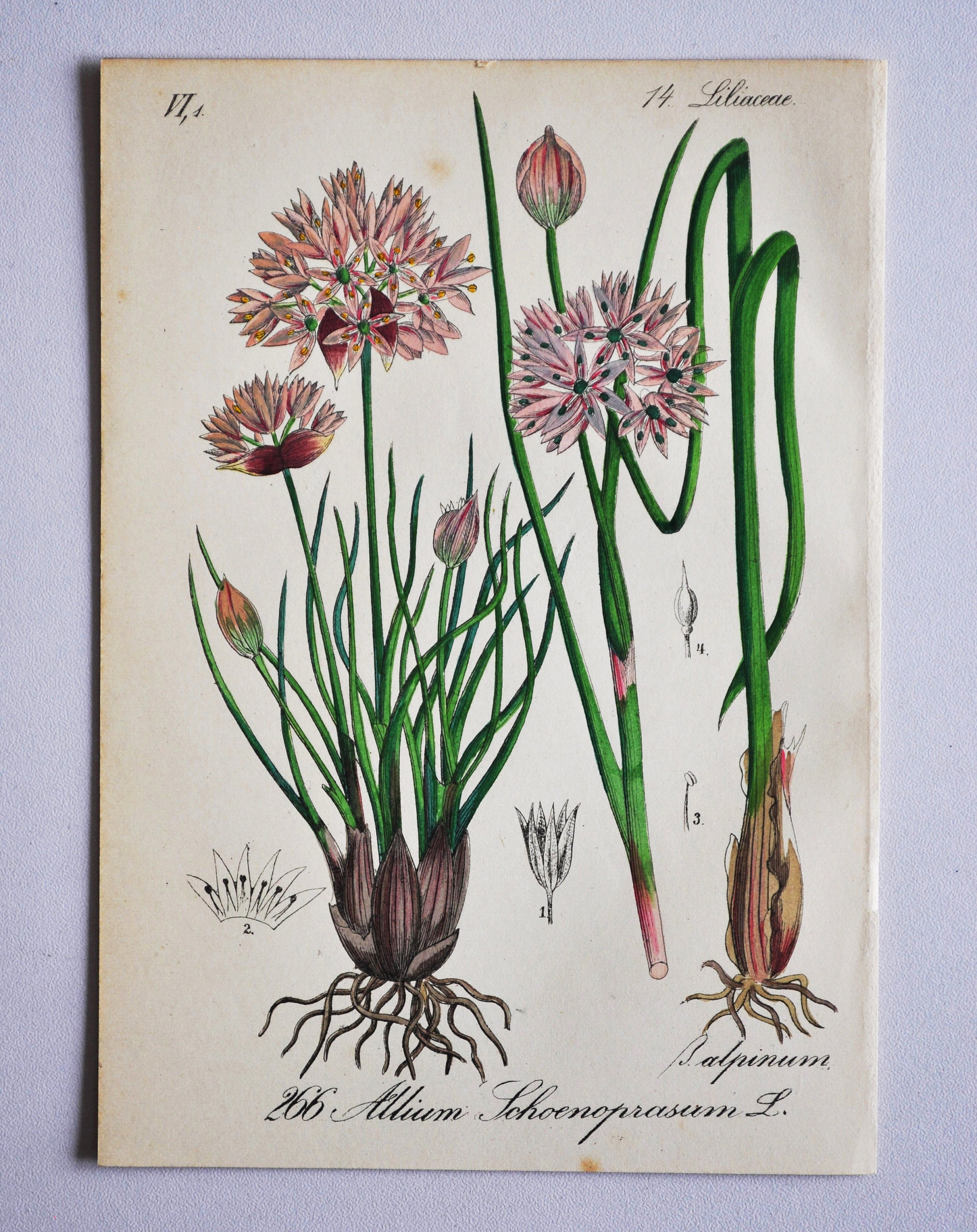The image features a detailed scientific illustration of a plant from the Liliaceae family, specifically labeled as Lilium Sheropresium or Allium showlifracium, with the annotation L266. The artwork, possibly a painting or digital graphic on a piece of slightly dirty paper, depicts the plant in various stages. The plant has green leaves and green stems, with roots that are brown and resemble those of an onion. At the top of the plant are multiple blossoms with light purple flowers, transitioning from buds to open petals that are light pink. In the center of the image is a prominent unopened flower bud. The text at the top left reads VI4, while the top right corner is marked with "1 4 Lilia K" and "14 Liliaceae" denoting the plant's classification. The illustration also includes diagrams numbered 1 through 4, showing different parts of the plant. The entire composition is set against a white background and annotated with cursive text that adds to its scientific presentation.